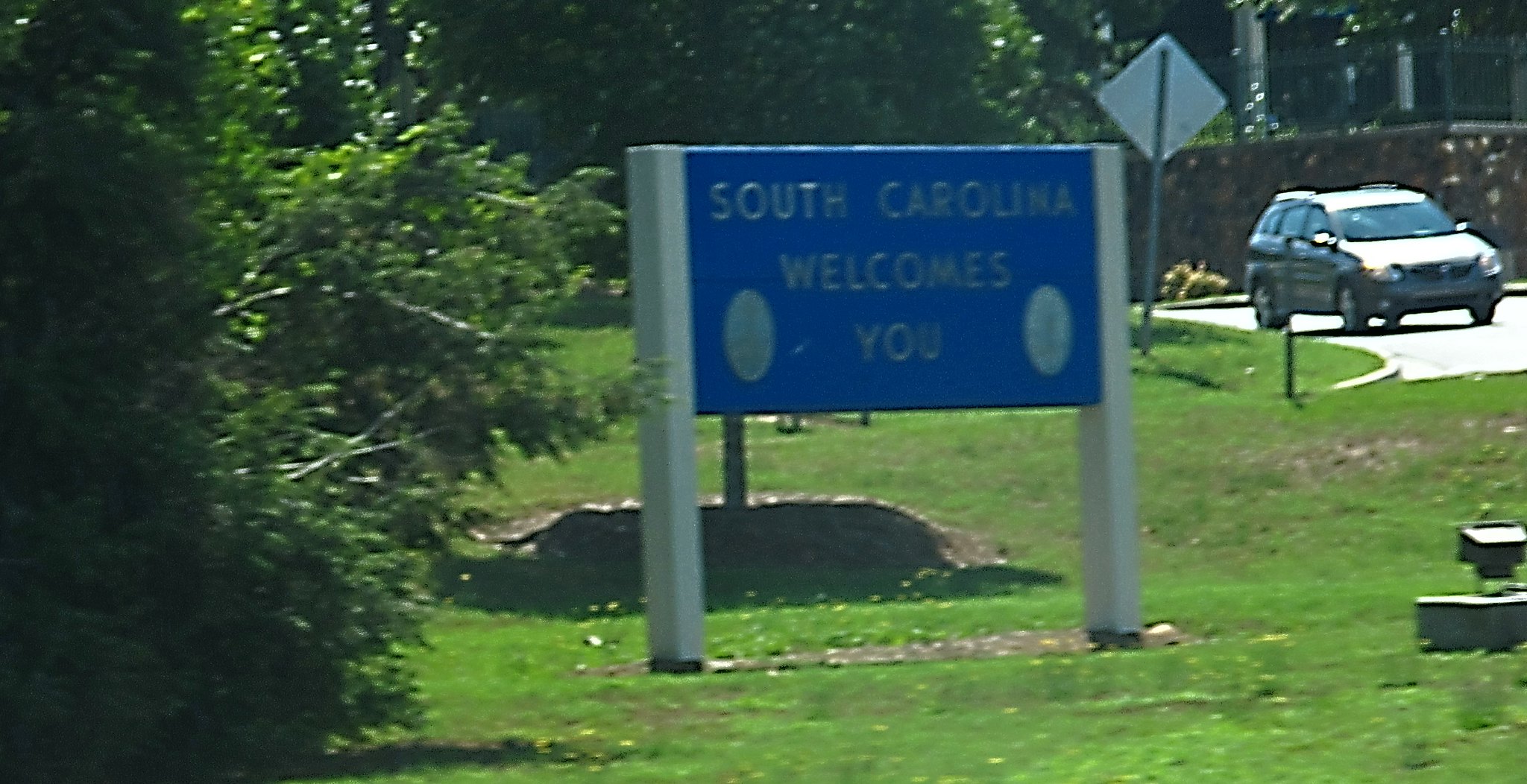In this picturesque outdoor scene, a vast expanse of lush green grass stretches out, leading the eye toward a dense cluster of trees on the right-hand side. Dominating the center of the image is a large, prominent sign. This sign stands tall on two sturdy white posts that rise from the ground all the way to the upper edge of the sign. The sign itself is a bold blue rectangle with inscriptions in contrasting white and blue lettering that read, "South Carolina Welcomes You." The sign also features two small, blank ovals positioned next to the word "You" for an additional touch of detail.

Adding to the narrative of the scene, in the upper right-hand corner, a crossover or small SUV can be seen driving along a road, lending a sense of movement and human presence to the tranquil, natural setting.